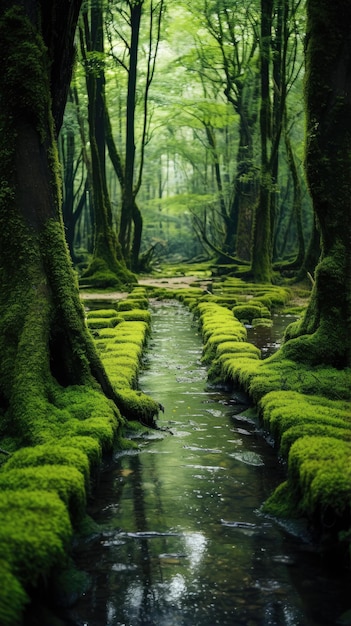This highly detailed painting captures a tranquil forest scene with a stream running through it, which looks almost like a photograph due to its realism. The stream is straight and rectangular, bordered by uniform, square-like rocks that are thickly covered in lush, green moss. The water surface is calm, adorned with small bubbles and reflective of both the surrounding forest and hints of sunlight filtering through the dense canopy above. Tall, deciduous trees with moss-covered bases line both sides of the stream, their thick branches and verdant leaves creating a leafy ceiling that allows only glimpses of the grayish sky. Shadows from these towering trees cast a serene, dim light over the scene. In the background, more tree trunks and bare rocks extend into the distance, enhancing the sense of depth. The overall scene exudes a peaceful, almost mystical forest atmosphere with the stream appearing to flow through a natural yet meticulously organized channel.